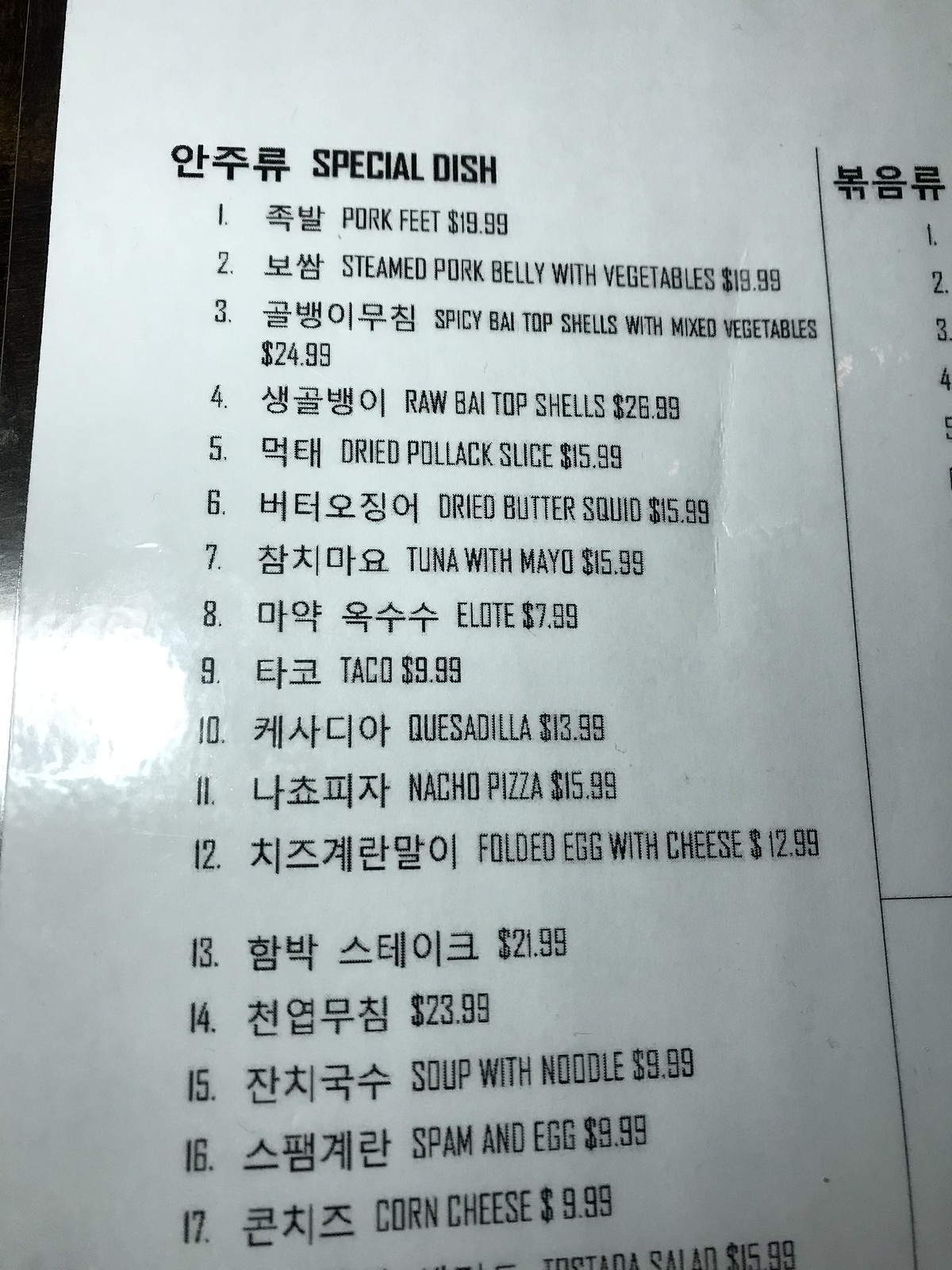Indoor color close-up photograph showcasing a portion of a menu set against a white background. The menu features 17 items, each listed with Korean characters on the left and corresponding English translations on the right. The menu is titled "Special Dishes" at the top, and each item is numbered sequentially from 1 to 17, followed by the dish name and its price.

The listed items are as follows:
1. Pork Feet - $19.99
2. Steamed Pork Belly with Vegetables - $19.99
3. Spicy Bi-top Shells with Mixed Vegetables - $24.99
4. Raw Bay Top Shells - $26.99
5. Dried Pollock Slice - $15.99
6. Dried Butter Squid - $15.99
7. Tuna with Mayo - $15.99
8. Elote - $7.99
9. Taco - $9.99
10. Quesadilla - $13.99
11. Nacho Pizza - $15.99
12. Folded Egg with Cheese - $12.99
13. [Dish name in Korean characters] - $21.99
14. [Dish name in Korean characters] - $23.99
15. Soup with Noodles - $9.99
16. Spam and Eggs - $9.99
17. Corn Cheese - $9.99

There is an additional column on the upper right side of the menu, partially visible, that contains Korean characters and the numbers 1 through 5.